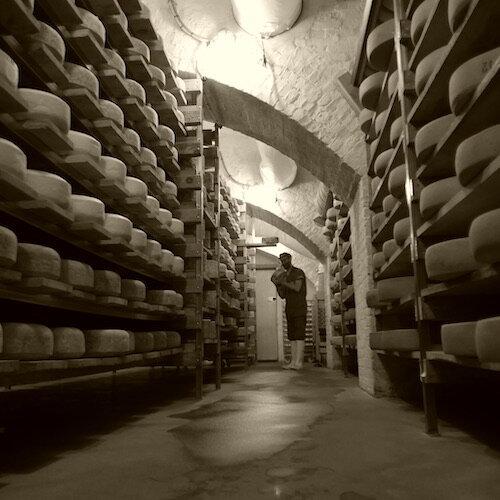In this photograph, there is a meticulously organized cheese aging cellar with white stone walls. The room features wooden shelves, filled from floor to ceiling on both sides, each holding dozens of large, foot to two-feet in diameter, white wheels of cheese. There are approximately eight shelves high on either side, forming a clear central pathway with a slightly wet floor. Toward the back of the room are four archways, two of which are prominently visible. A man stands under one of these archways, facing left and holding one of the cheese wheels. He is dressed in a short-sleeved dark shirt, dark pants tucked into knee-high white rubber boots, and a captain-style hat. His face is blurred, but a beard is visible. The photograph is illuminated by lights from the ceiling, despite there being no other people, animals, or visible writing in the image. The overall ambiance is that of a detailed, sepia-toned or possibly color image capturing the essence of traditional cheese aging processes.